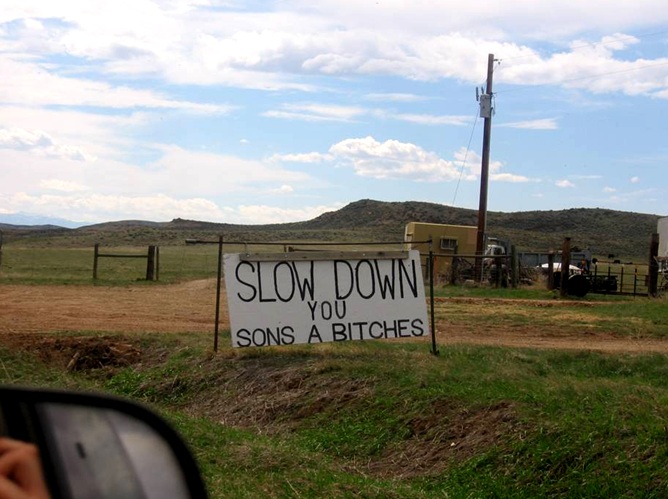The image captures a scene from a rural countryside, likely a farm, with a touch of humor and seriousness. Taken from inside a car, evidenced by the partial view of the passenger side rear view mirror in the bottom left corner, the photograph prominently features a white sign with bold black text that reads, "SLOW DOWN YOU SONS OF BITCHES." The sign, supported by three black poles—two vertical and one horizontal—stands beside a dirt road that winds through lush green grass and into the background of expansive green fields and rolling hills. The sky overhead is a serene blue, adorned with fluffy white clouds. In the distance, a yellow vehicle and what appears to be an electric pole suggest the presence of farm-related activities or a junkyard. The overall scene conveys the need for drivers to reduce speed in this tranquil, animal-inhabited area, combining a rustic charm with a straightforward message.